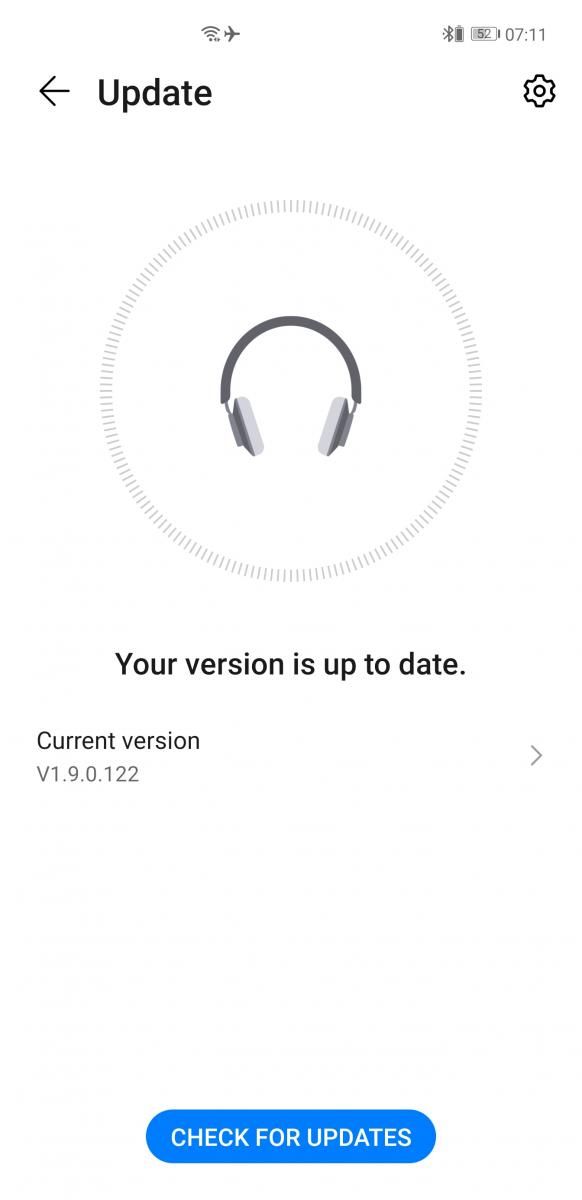The image appears to be a screenshot from a headphones app. At the top right corner, the current time is displayed as 7:11. Adjacent to the time, on the left, is a horizontal battery symbol indicating a battery level of 52%. Further left, there is a Bluetooth symbol. Centrally located at the top is a full-strength Wi-Fi icon, flanked by a small airplane mode symbol to its right. Below these icons, prominently in the center, is the word "Update" accompanied by a left-pointing arrow. An empty space follows to the right of "Update," culminating with a gear icon indicative of settings.

Dominating the central portion of the image is a visually striking circular image of headphones. The headphones feature white ear cups contrasted by a black headband. Beneath the image is the reassuring text "Your version is up to date," followed by detailed version information: "Current version: version 1.9.0.122." An arrow points to the right from this text, separated by an empty space on its left.

At the bottom of the image, a blue rectangular banner vividly displays the words "Check for updates" in white text.